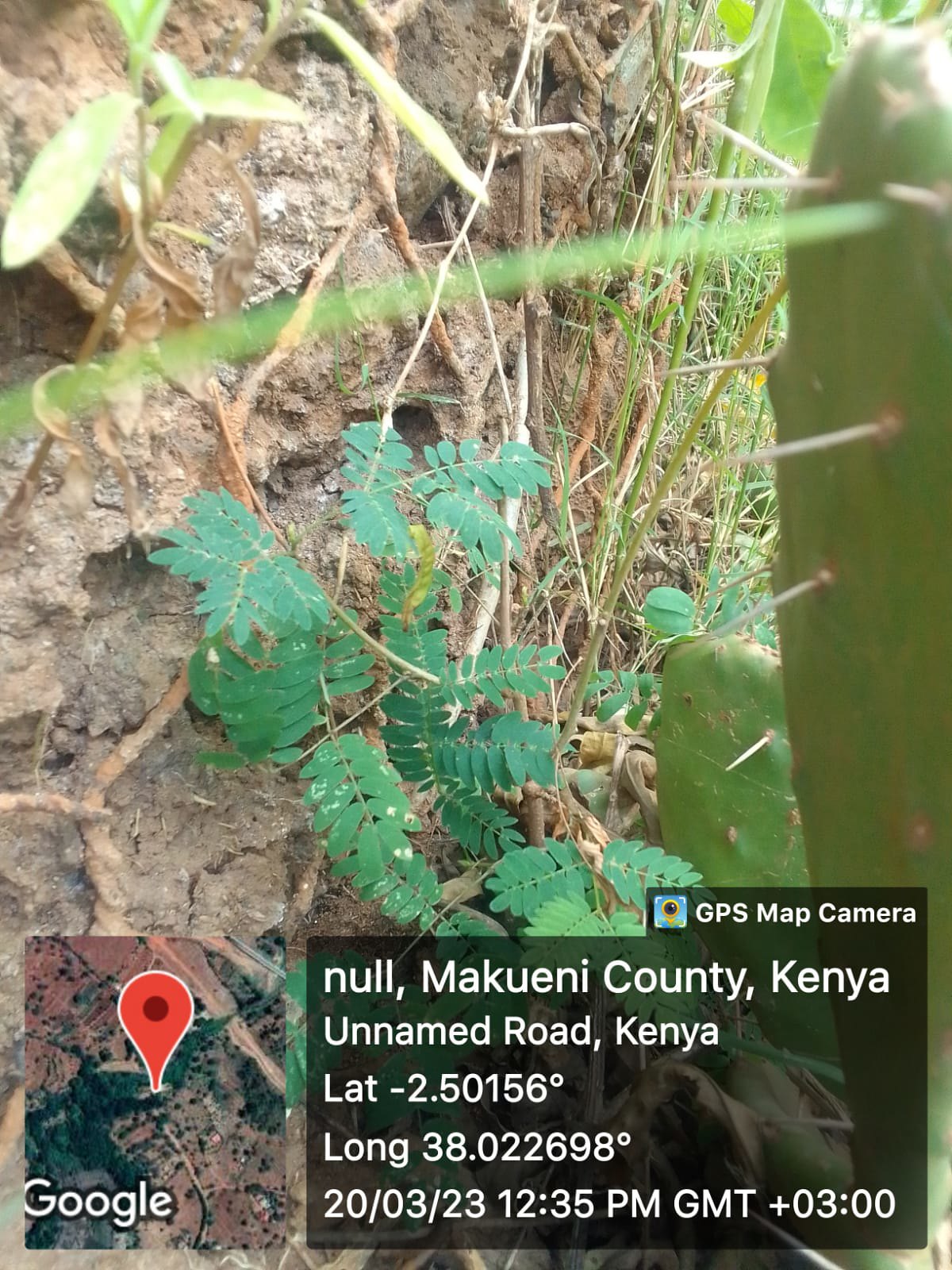This detailed photograph captures an aerial view of an expansive arid landscape showing intermittent patches of greenery. In the bottom left corner, a map with a marker pinpoints the photograph's location. In the image's foreground, a vibrant green fern emerges from a rugged rock surface. Adjacent to the fern, a cactus with multiple sharp white needles stands resilient. The bottom right of the image features a partially transparent black rectangle with white text, providing contextual information: "null, Makwani County, Kenya, unnamed road, Kenya, LAT -2.0156 degrees, LONG 38.022698 degrees, 20/03/2023, 12:35 PM GMT +03:00." The scene is complemented by the additional detail from the opaque black frame, which includes a note that this photo was taken using a GPS map camera. The location's specificity and the photograph's natural elements suggest a serene yet rugged environment, possibly within a park in Kenya.